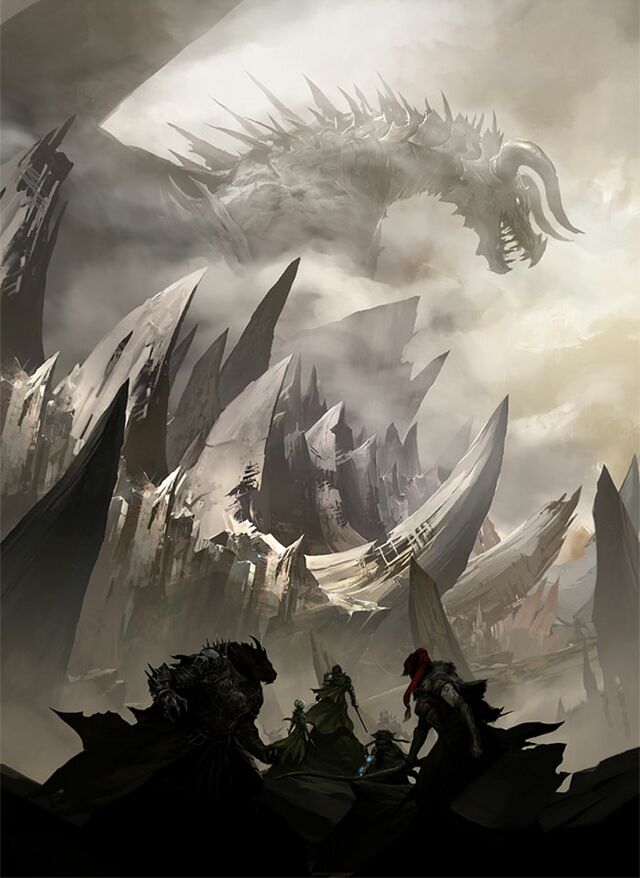In this intricate black and white illustration drawn with shades of gray, a grand and imposing dragon dominates the scene, looming menacingly above a jagged, rocky mountainscape. The dragon, cresting over sharp, fang-like peaks, flaunts an array of spiky spines running from its head down its back, along with pronounced horns and a gaping mouth filled with gnarly, sharp teeth. Clouds wisp around the monstrous creature, accentuating its size and ferocity as it gazes leftward. Below, in stark black relief against the pale, jagged mountains, a group of indistinct, shadowy figures—likely determined, armed warriors on horseback—stand dwarfed by the scene. In the foreground, these heroes appear poised, possibly ready to confront a smaller dragon to the left, their faces obscured but their resolve palpable, creating a tense, climactic moment set in a desolate, rugged fantasy landscape.